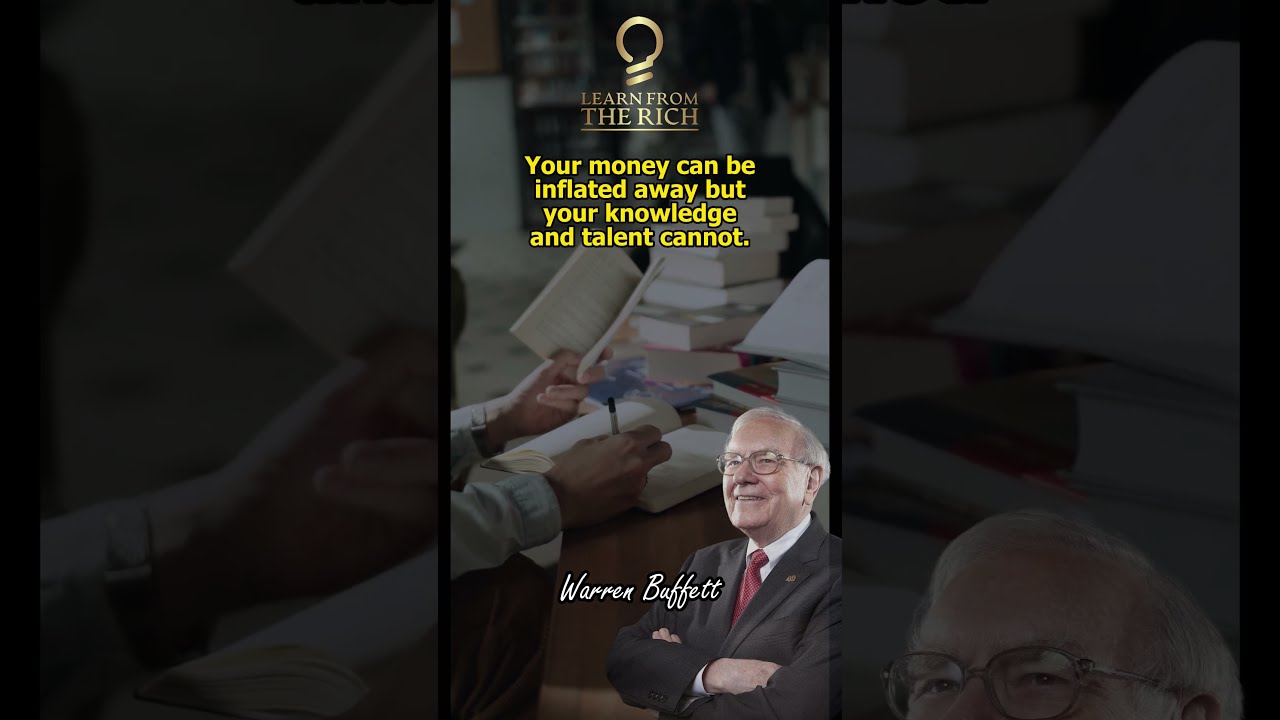The image presents Warren Buffett at the center, smiling with his arms crossed. He is dressed in a dark suit, white shirt, and red tie with glasses on. His name, "Warren Buffett," is written in white letters across his chest. The page is divided into thirds, with the left and right thirds showing blurred, enlarged segments of the central image. The background features a man in a white shirt sitting at a desk, writing with a pen in his right hand, surrounded by books. At the top center, against this background, there's a logo resembling a light bulb, and below it, in gold letters, it says "Learn from the Rich." Underneath, in yellow lettering, the text reads, "Your money can be inflated away, but your knowledge and talent cannot."